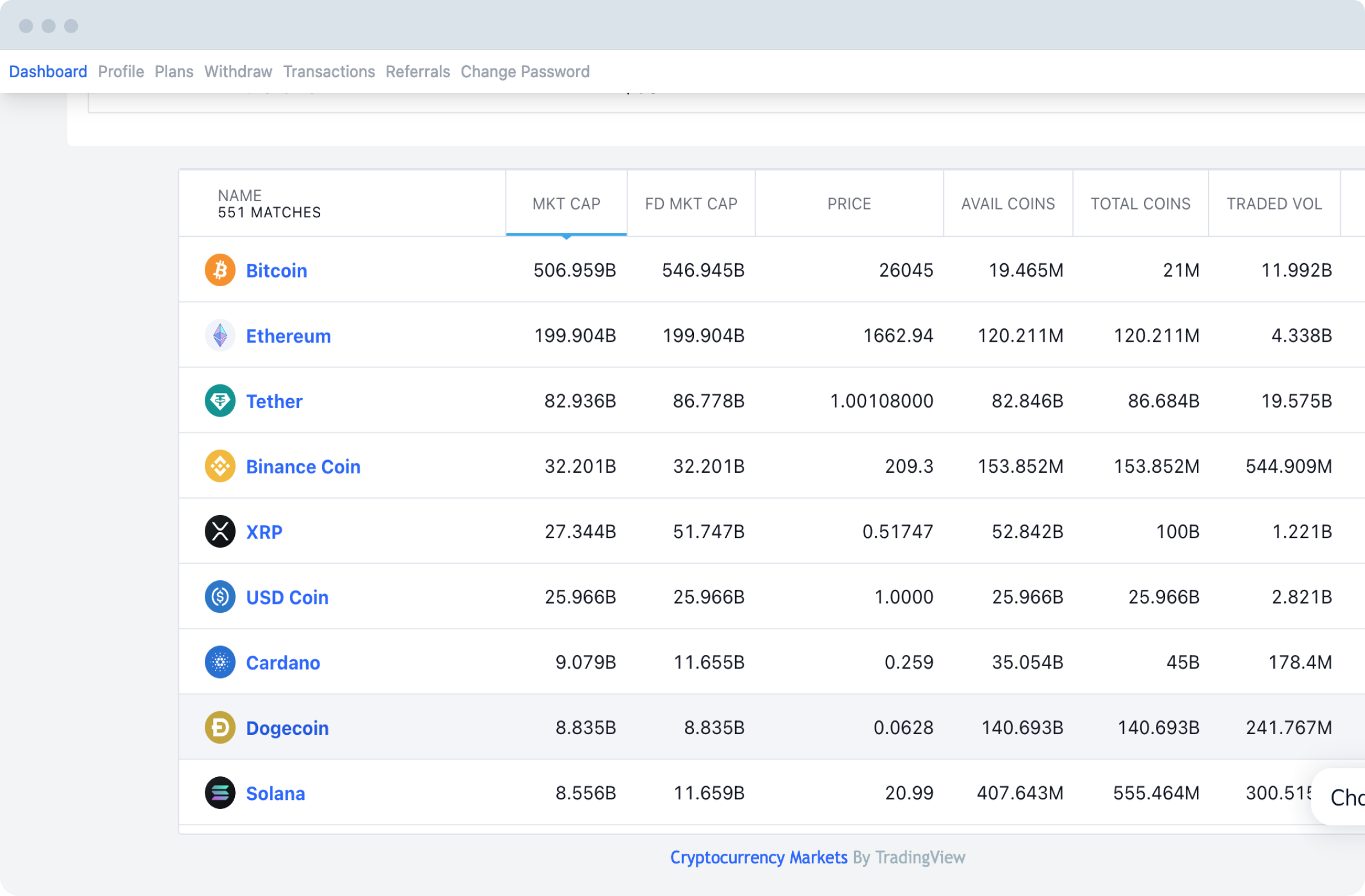The home screen of a computer program is displayed, featuring a clean, white background. At the top, a gray horizontal bar spans the width of the screen with three darker gray dots aligned in the upper left corner. Just below the gray bar, the word "Dashboard" is prominently displayed in blue text. 

Below the "Dashboard" header, a vertical menu lists several options in dark gray text: "Profile," "Plans," "Withdraw," "Transactions," "Referrals," and "Change Password." 

In the main content area, the text "Name" along with "551 matches" is displayed in black. Following this, detailed information about Bitcoin is provided, starting with "Bitcoin" in blue text, then "Market Cap" at 506959B, "FD Market Cap" at 546945B, "Price" at 260.45, "Available Coins" at 19.465M, "Total Coins" at 21M, and "Traded Volume" at 11.992B. 

On the left side, a list of other cryptocurrencies is presented in blue text: "Ethereum," "Tether," "Binance Coin," "XRP," "USD Coin," "Cardano," "Dogecoin," and "Solana."

At the bottom center of the screen, "Cryptocurrency Markets" is shown in blue text, with "By Trading View" written in dark gray just below it.